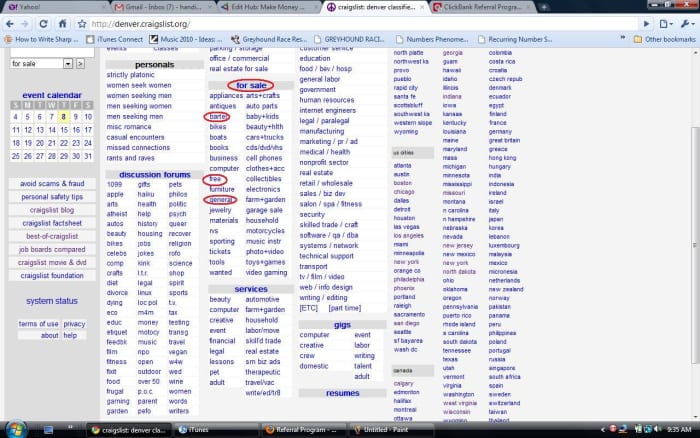Screenshot from a computer displaying a web browser with multiple tabs open including Yahoo, Gmail, Edit Hubs, and Craigslist, with the latter currently selected. Below the toolbar, there's a referral link to ClickBank. To the left of the URL bar, which reads 'Denver.Craigslist.org', are the back, forward, refresh, and home buttons.

The browser's bookmarks toolbar includes links related to numbers, greyhound racing, and iTunes connections, among others. The Craigslist page prominently features its characteristic vertical menu on the left, consisting of an event calendar, search fields, and options for fact sheets, avoiding scams, and safety tips.

On the right side, there is a myriad of text links categorized under sections such as personals, where options include 'platonic' and 'women seeking men', as well as discussion forums with around 60 categories. The 'for sale' section, along with 'barter', 'free', and 'general', are all circled in red pen, indicating significant interest. Additionally, the page offers sections for services, gigs, resumes, and countless other categories typical of Craigslist's extensive directory.